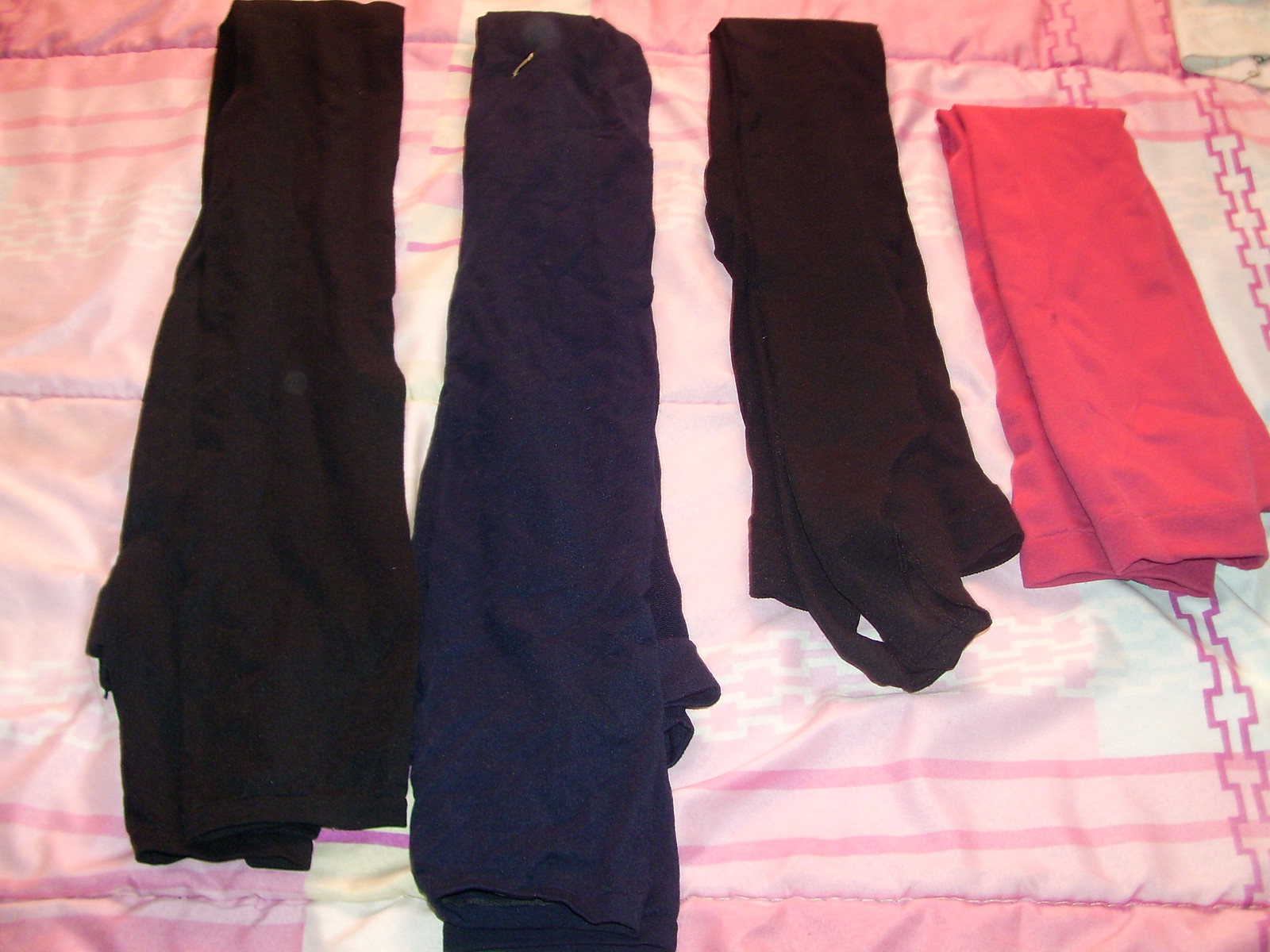In the image, a vibrant, pink-patterned bedspread, adorned with various shades of pink from light to dark, covers a bed. This bedspread features a soft texture and a geometric design. Laid out in an orderly fashion on the bedspread are four pieces of clothing, appearing to be women's pants or leggings, carefully folded in half. The garments are arranged from left to right in the following order: black, dark navy blue, black, and hot pink. The hot pink pair is notably smaller than the others. Additionally, there is a coral-colored towel amidst the neatly positioned clothing, suggesting that someone might be preparing to pack for a trip. The bedspread is slightly wrinkled, adding a casual touch to the meticulously laid out items.